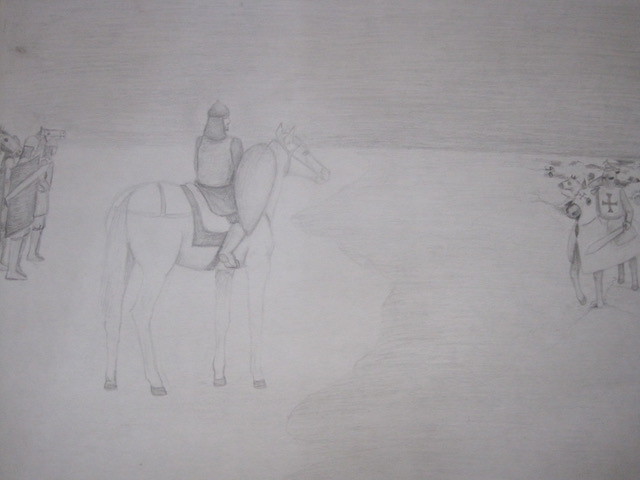This detailed pencil sketch depicts a medieval scene with two armored knights on horseback. The upper third of the paper features intricate shading, which sets a dramatic backdrop for the foreground action. The first knight is mounted on a horse adorned in traditional knight's caparison and wields a sword. This knight is depicted wearing full body armor, with a prominent chest piece bearing a cross. The second horse is significantly taller, with long, sleek legs and is depicted without any decorative coverings, only wearing a saddle and bridle. The knight riding this taller horse is turned away from the viewer, yet the armor detail is evident, adding to the sense of realism in the sketch. The meticulous detail in the armor and horses, combined with the atmospheric shading, gives the drawing a powerful and evocative medieval feel.